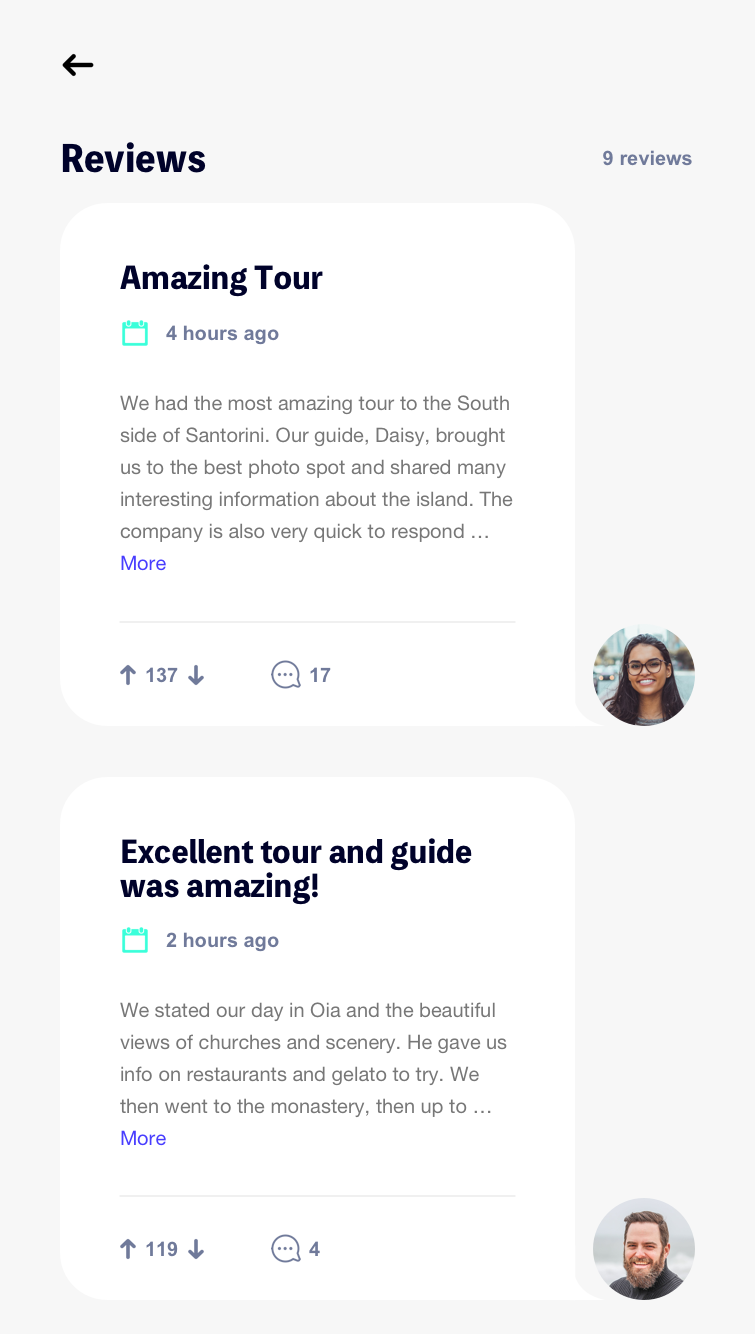This vertical rectangular image set against an off-white background contains a variety of review details and user interactions. 

At the top left corner, a bold black arrow points to the left, indicating navigation, with the word "Reviews" in bold black font next to it. To the right, the number "9" signifies the number of reviews. 

Beneath this is a vertical rectangular box with rounded corners, displaying the title "Amazing Tour" in bold black font on the left-hand side. Underneath, a small green icon is present, followed by the text "Four Hours Ago" in gray font. The review itself begins in gray font, stating, "We had the most amazing tour to the south side of Santorini. Our guide, Daisy, brought us to the best photo spot and shared many interesting information about the island. The company is also very quick to respond..." The word "More" appears in purple font at the bottom left of this review.

Further down, the page shows the numbers "137" with an up arrow to the left and a down arrow to the right, indicating the review votes, alongside a talking bubble icon with the number "17" representing the comments. To the far right on the off-white background appears a picture of a woman with dark hair and glasses.

Below this, another white vertical rectangle with rounded corners is present. This review is titled "Excellent Tour and Guide was Amazing!" in bold black font. A small green rectangle under the title is followed by text in gray font, "Two Hours Ago," indicating the time of the review. The review description continues in gray font, "We started our day in Oia with its beautiful views of churches and scenery. He gave us info on restaurants and gelato to try. We then went to the monastery, then up to..." The word "More" appears again in purple font below this review.

At the bottom of this review, the number "119" is displayed with an up arrow to the left and a down arrow to the right. A speaking bubble icon with the number "4" is next to it, representing the number of comments. Finally, in the off-white area, there is a small circular image of a man with a mustache and beard.